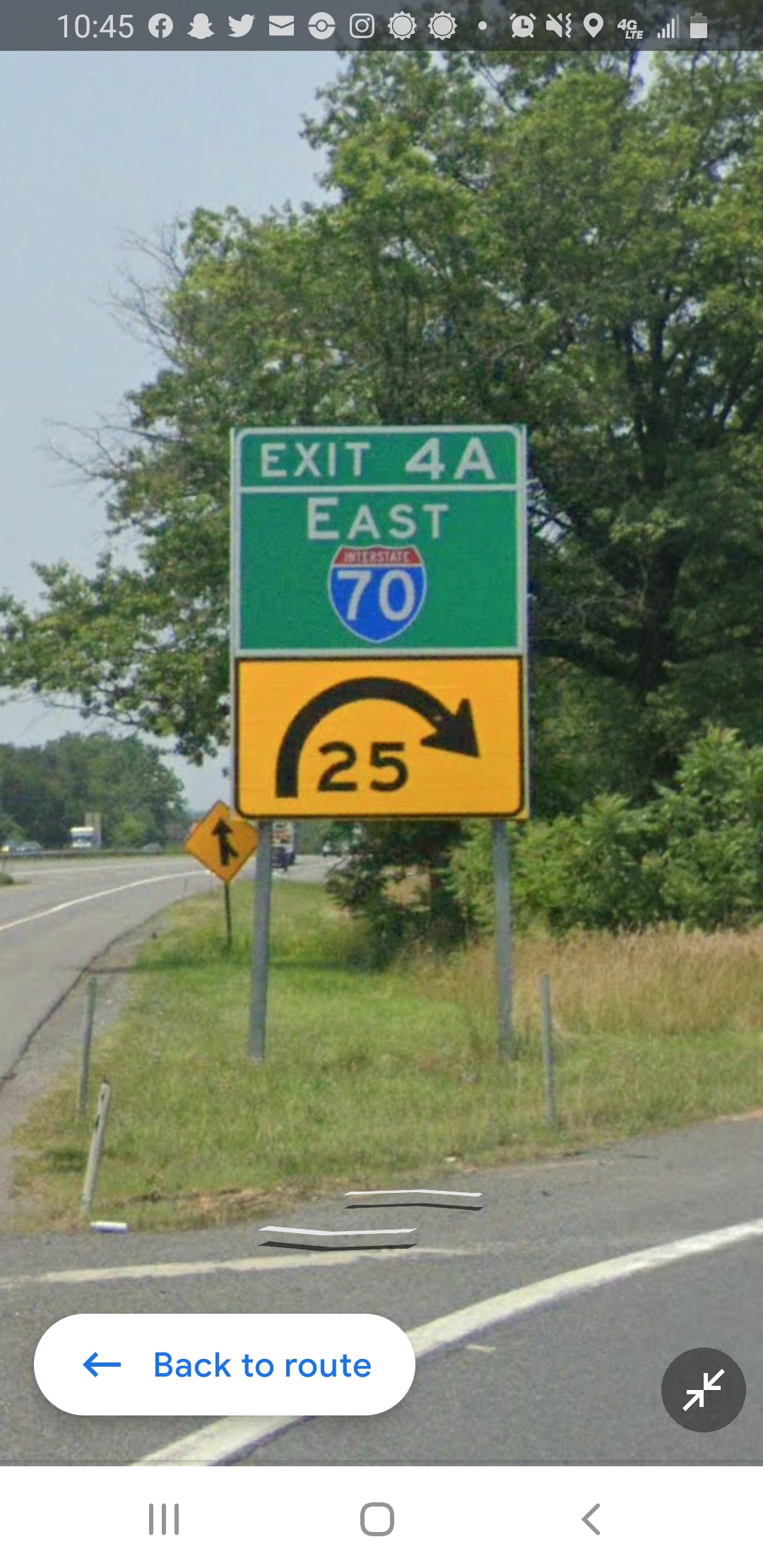This photograph, likely taken from the windshield of an automobile on an exit ramp off East Interstate 70 in the United States, captures the green exit 4A sign with white lettering supported by two metal posts. Below the exit sign is a yellow caution sign displaying a black arrow curving right and a speed limit of 25 mph. The shot includes part of the exit ramp and showcases another diamond-shaped merge sign visible behind a large tree in the background on the upper right. The foreground features two white angled pieces of material, possibly wood or plastic, in the vicinity of the exit sign. The image was taken on a clear sunny day with no clouds in the blue sky, and additional details indicate it was shot on a cell phone, as evidenced by the black bar at the top showing the time (10:45) and various app icons.